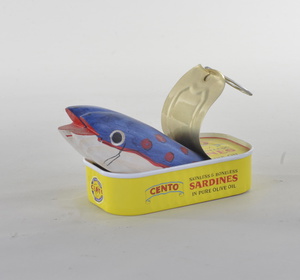In this square photograph with a featureless white background, the focal point is a yellow can of Cento brand sardines in pure olive oil, prominently positioned at the center. The can features a gold-colored ring-pull lid that has been pulled back about two-thirds of the way, revealing its contents. Emerging from the can is a toy fish, resembling a fishing lure or possibly a stuffed animal sardine. This whimsical fish toy has a blue top adorned with red polka dots, a white belly, and vivid details including an open mouth with a red interior and a single visible black eye. The fish is oriented as if facing west, playfully appearing to escape from the can. The label on the can displays "Cento" in bold letters along with "sardines in pure olive oil" in red text, although some smaller text is not clearly legible. The surreal and humorous nature of the image is accentuated by the oversized fish that contrasts with the expected contents of the sardine tin.